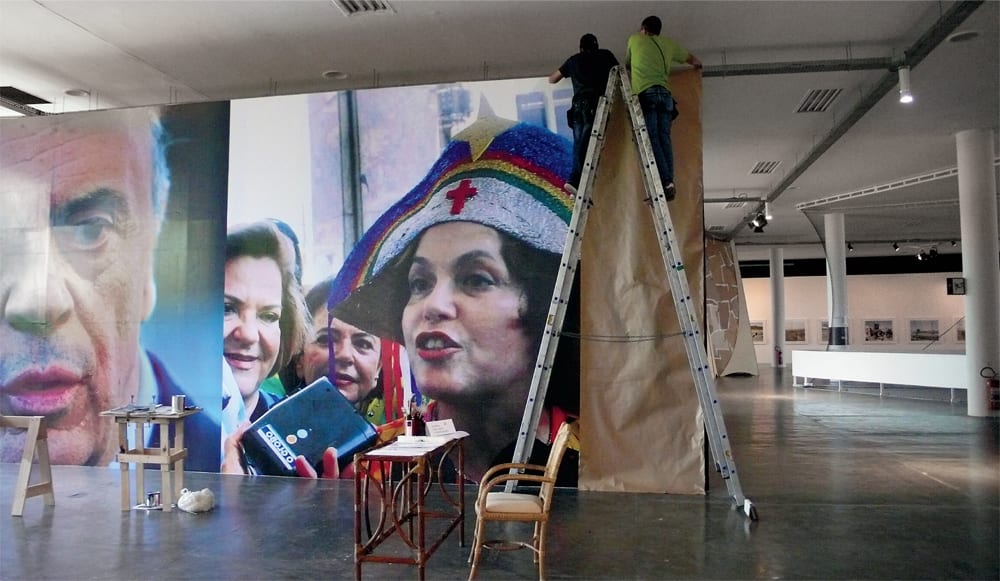This photograph captures a detailed scene of an art gallery during the installation of a large photographic mural. Positioned at the center, two men are standing on a tall, silver ladder. The man on the right wears a bright green t-shirt and blue pants, while the man on the left is clad in a dark blue t-shirt and dark blue jeans. They are affixing massive images to the walls, which stretch from the white ceiling down to the polished gray concrete floor.

To the left of the men, a large close-up portrait of an elderly man with short gray hair and a serious expression is visible. He dons a dark blue suit jacket over a white shirt. Adjacent to his image is a vibrant photograph of a woman with short black hair, her head adorned with a distinctive multicolored hat. The hat boasts a white front area featuring a red cross and three lines in green, yellow, and red, topped by a larger blue band with a yellow cross. Her mouth is slightly open as if she is speaking. Two women in the background appear happy, adding life to the gallery scene.

In the foreground, there is a dark brown table with a light brown chair positioned in front of it, alongside an additional small wooden table that holds some instruments. There's also a visible sawhorse nearby. The far wall showcases a collection of six or seven framed photographs or paintings, adding to the artistic ambiance of the space. The room itself features pillars and light fixtures, enhancing this intricate depiction of ongoing artistic labor.